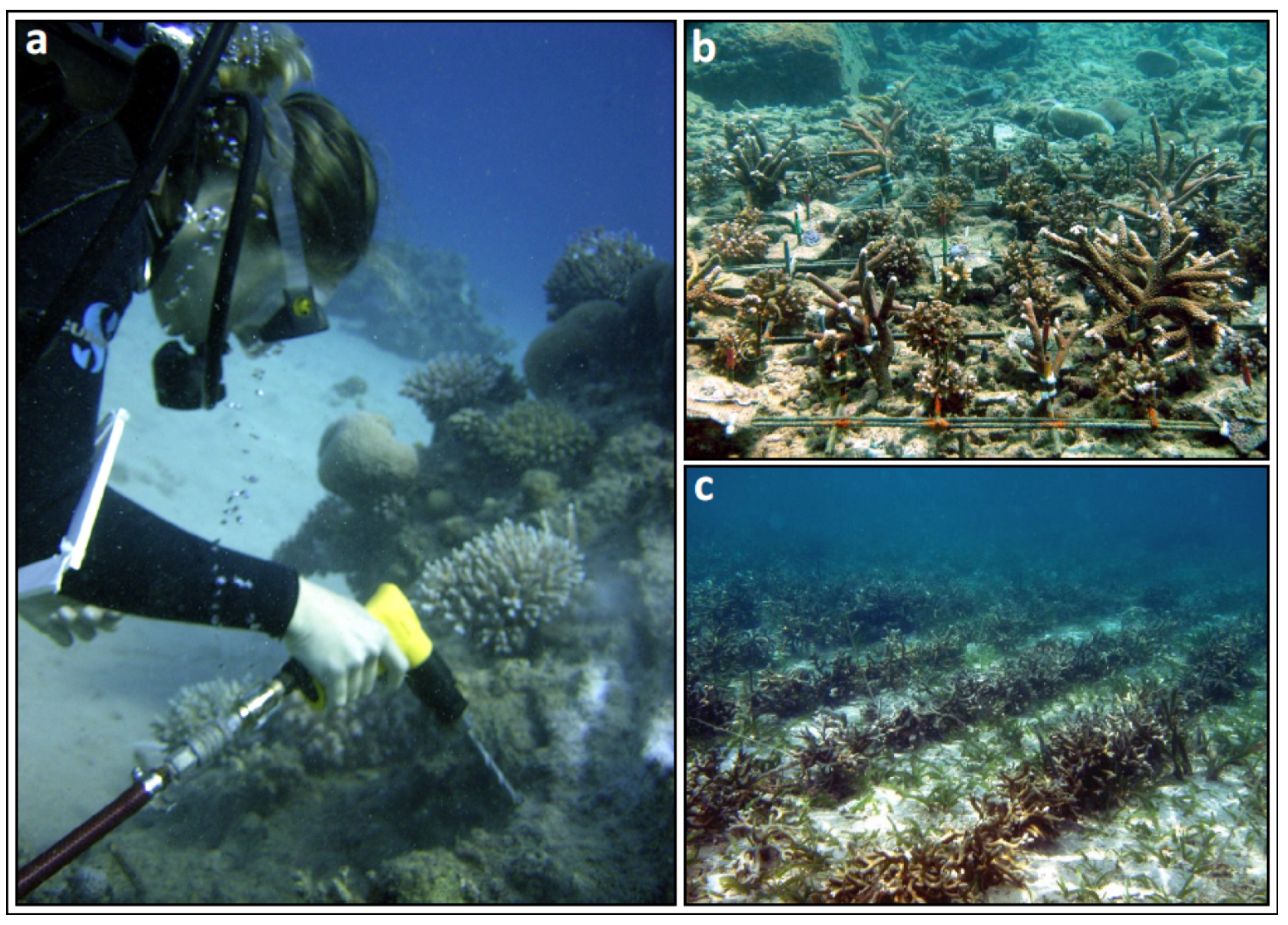The image consists of a collage with three frames labeled A, B, and C. The left frame, labeled A, features a woman deep-sea diving, dressed in a black wetsuit and wearing a breathing apparatus with goggles. She has medium blonde hair pulled back and is underwater, surrounded by bubbles. The diver, a white woman, is holding a yellow and black drill-like device with a hose, pointing it towards the ocean floor, which is dotted with coral and sea anemones. Frames B and C, on the right, display underwater vegetation that appears to be cultivated in organized rows, suggestive of an underwater farm or habitat. These frames provide different perspectives of the aquatic plants, which range from well-maintained vegetation to ridged formations, possibly sea urchins or coral.